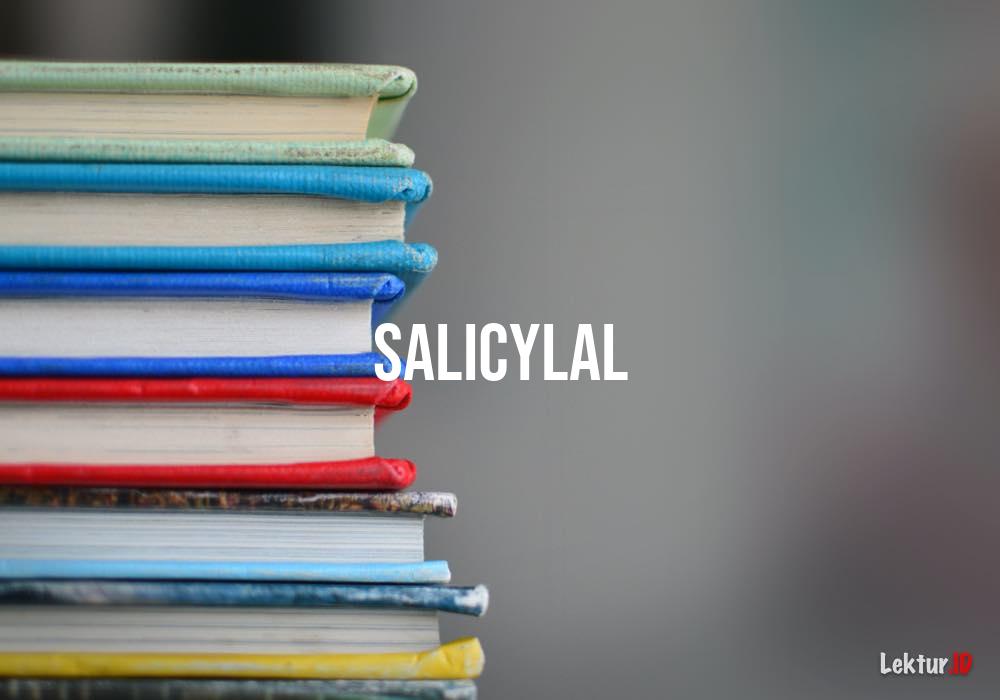Against a varying gray backdrop, a stack of thin, hardcover books is positioned on the left side of the image. The books are arranged in descending order of color: light green, light aqua blue, royal blue, medium red, a split binding of brown and light blue, medium blue, yellow, and a barely visible green-blue at the bottom. Prominently centered is a bold word in all capital white letters, "S-A-L-I-C-Y-L-A-L." In the lower right corner, a small logo reads "L-E-C-T-O-R" in white, followed by "J-D" in red.